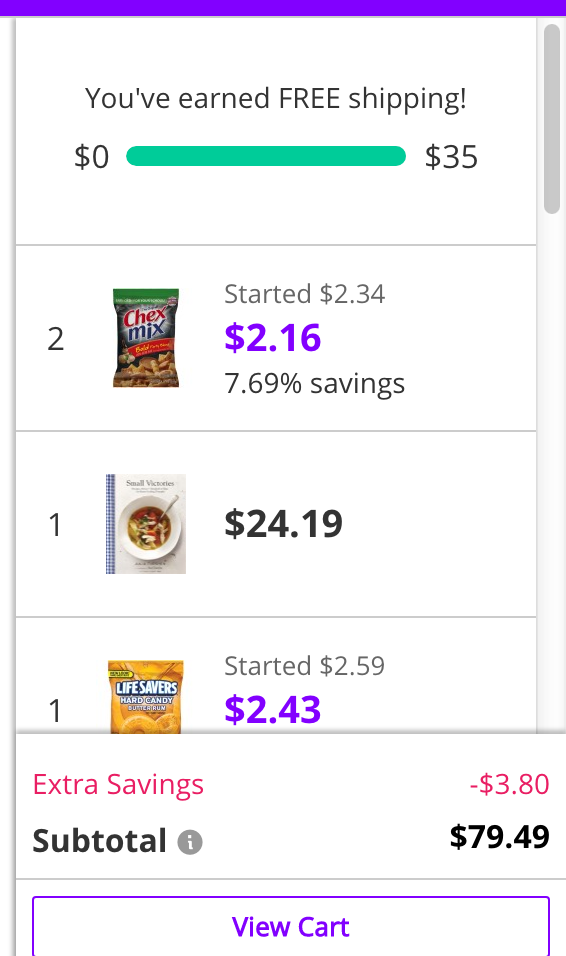**Detailed Caption:**

The image shows a screenshot of a shopping cart page, likely from a mobile app, featuring a distinctive purple bar at the very top. This bar indicates the shopper's progress towards earning free shipping, showing "$0" on the left and "$35" on the right, with a green bar almost completely filled between them.

Below this, the cart includes several items with detailed pricing information:

1. **Chex Mix** - Originally priced at $2.34, with a discount, it is now $2.17, reflecting a savings of 7.69%.
2. **Soup** - Priced at $24.19.
3. **Lifesaver Candies** - Originally priced at $2.59, now available for $2.43. There's also an extra savings of $3.80 displayed in red.

Further down, the cart shows a subtotal of $79.49. At the bottom, there is a purple-outlined button with purple lettering that reads "View Cart."

The right side of the image features a visible scroll bar, suggesting more items might be listed if scrolled down. The overall layout and interface elements, such as the progress bar and buttons, hint that this could be a shopping cart page from a service like Instacart or Walmart.